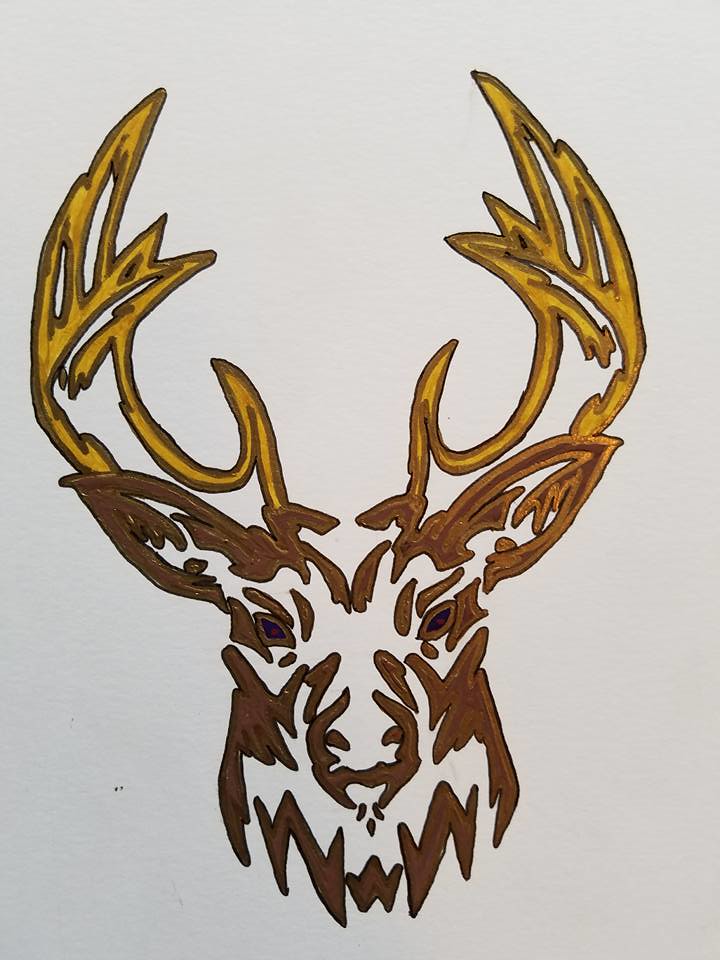This image showcases an artwork of a deer, specifically a stag, rendered with pencil, colored pencil, or pen. The portrait focuses on the head, neck, and antlers of the deer. The stag is depicted in varying shades of brown; darker brown is used for the inner features, while a lighter brown outlines these details. The antlers, which extend upward and curve gracefully with a feather-like quality at their tips, are tinted gold and outlined in brown. Unlike a fully colored illustration, this artwork includes strategic white spaces that accentuate the nose, eyes, and other intricate details, thereby adding depth to the portrayal. The deer’s ears extend diagonally from its head, adding to the realistic yet somewhat stylized representation. The overall effect suggests that the piece is the work of a young artist—perhaps a talented teenager. The drawing successfully captures the essence of the deer, blending both artistic skill and simplicity.